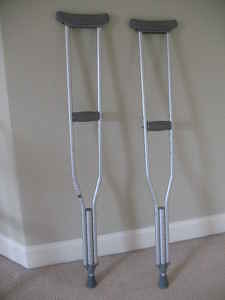The photograph depicts a pair of standard aluminum crutches positioned side-by-side, leaning against a light gray wall. The wall features a white baseboard at the bottom, with its corner visible in the lower left of the image. Both crutches are identical in height and design, with padded gray tops designed to fit under the user's armpits and padded gray handles midway down for hands. The tips of the crutches are covered in a lighter gray rubber material that makes contact with the floor. The flooring is a gray-colored carpet, contrasting with the white baseboard and the light gray wall. Despite being a low-resolution, pixelated photo, the details of the crutches' functional features and the room's color scheme are clearly discernible.